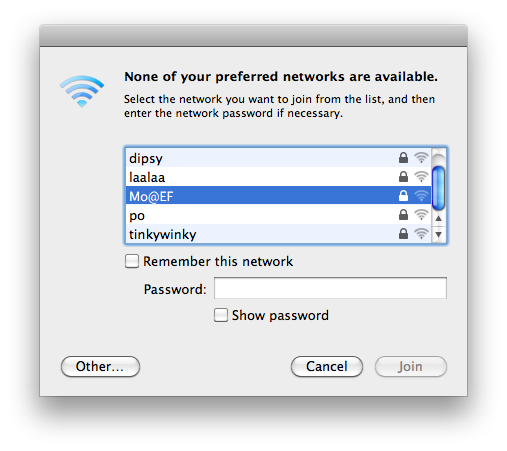The image depicts a grey pop-up window for connecting to the internet or Wi-Fi on an Apple device. The window features a darker grey band at the top, next to which is an internet icon. Below it, bold text states, "None of your preferred networks are available." Instructions are provided: "Select the network you want to join from the list and then enter the network password if necessary." The main body of the window contains a blue-highlighted list of various Wi-Fi networks, including names like "Moo GF" and "Tinky Winky," each marked with a lock icon to indicate they require a password. Beneath this list, there is a password entry field accompanied by a checkbox option to show the entered passwords. At the bottom of the popup are three buttons labeled "Other," "Cancel," and "Join." The entire interface is colored in shades of grey, white, and royal blue, with the network signal strength indicated at the top. This detailed digital representation is viewed straight on, likely on a laptop screen, with no indicators of the time of day.